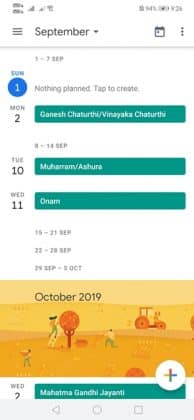In this image, we see a screenshot of a calendar app displaying the month of September 2019. At the top left, the title "September" is prominently displayed, with a three-line menu icon beside it. To the right, there is a small calendar icon and a three-dot menu symbol. As we move down the calendar, we notice the days are listed with specific annotations. 

On Sunday, the 1st, it states "Nothing planned. Tap to create." Monday, the 2nd, has an event marked, seemingly in another language. Tuesday, the 10th, also shows a scheduled event. Wednesday, the 11th, features the event "ONAM." These are the main dates highlighted in the month view.

Towards the bottom, the calendar transitions to October 2019, with a charming illustration depicting an outdoor scene. It features people in a field, one person on a ladder picking fruit from a tree, and a tractor in the background. Beneath this, although partially cut off, we can see the beginning of October with "Wed 2" marked by a green rectangle, indicating another scheduled event.